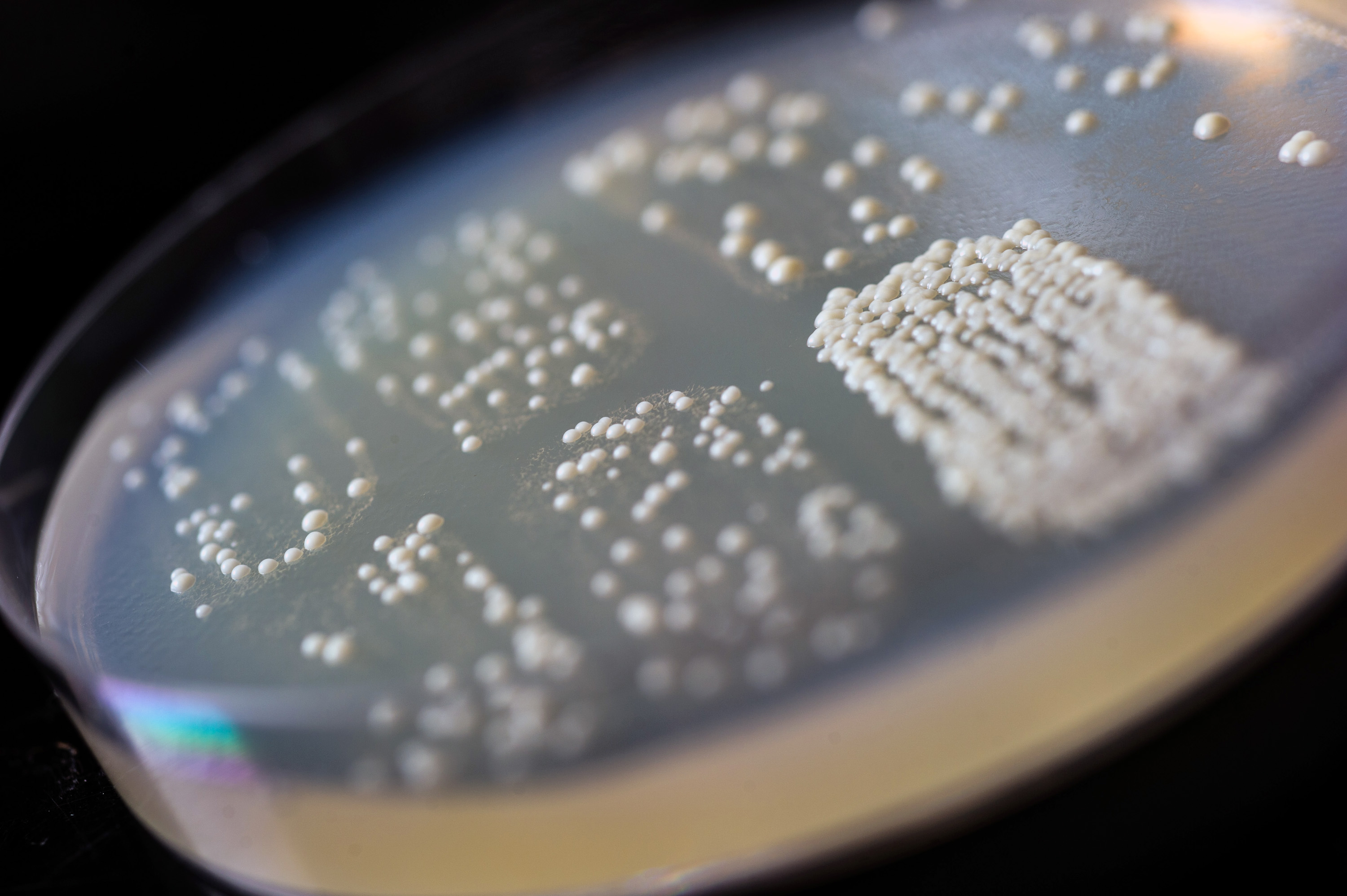The image depicts a close-up view of a Petri dish set against a black background, positioned diagonally with its upper edge pointing toward the upper right corner. The surface of the dish is green, dotted with small white bumps or specks, which represent bacterial colonies. These white dots are sparsely distributed at the top, but about a third of the way down, the pattern becomes denser and forms two square shapes filled with white dots, one densely populated and the other more sparse. As you move further down, two more sets of similar square shapes appear, and at the very bottom, there are another two squares with very few white spots. The dish appears to have a glass border, segmenting it into eight sections, each varying in the density of the white bacterial colonies.